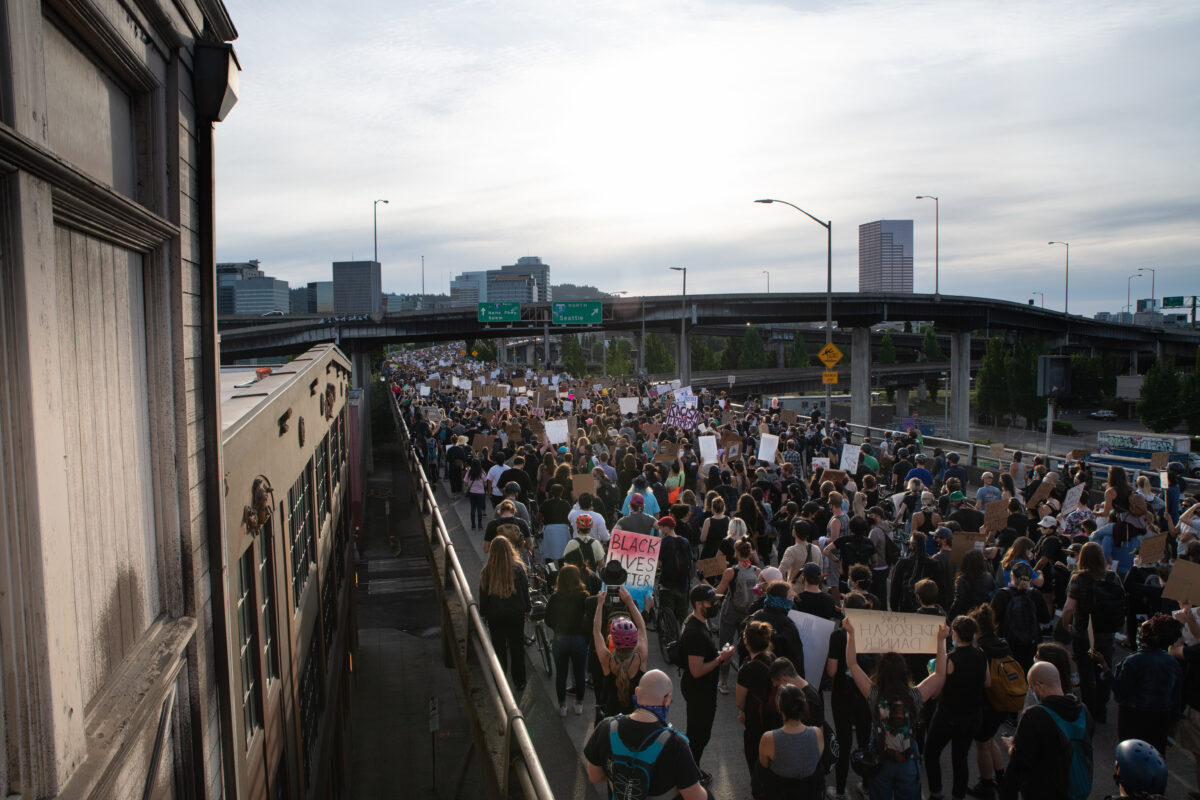This powerful photograph captures a Black Lives Matter protest on an elevated road, densely packed with people clad predominantly in black clothing and masks. The protesters fill the roadway, standing shoulder to shoulder, with several holding up signs, including one prominent sign in the lower part of the frame with red, white, and blue stripes adorned with the words "Black Lives Matter" in bold black text. The road stretches from the center left toward the bottom right, bordered by metal fences on either side, clearly obstructing the usual flow of traffic.

To the left of the frame, a beige stone or concrete building with bluish windows adds an urban touch. In the distant background, a striking skyline of blocky, glassy buildings emerges, with a notably taller glass structure standing out to the right. Directly above the protesters and in front of the skyline, a bright green highway sign with white text and arrows is clearly visible. The sky hangs heavily with streaks of white to light gray clouds, allowing slivers of sunshine to peek through, casting a muted light over the scene.